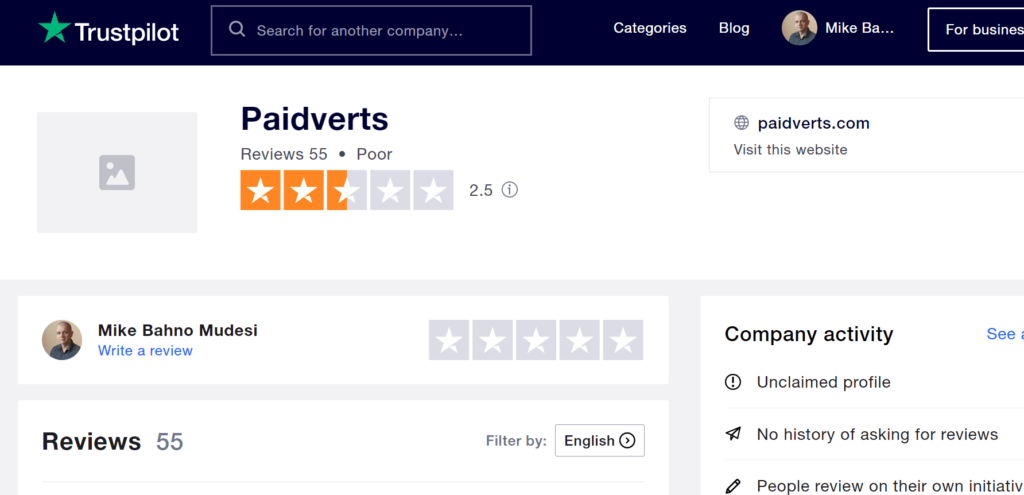A detailed screenshot from the Trustpilot website displaying a profile page for the company PaidVerts. The top section features the Trustpilot logo with a green star in the upper right-hand corner and a black background. Below, there is a search bar labeled "Search for another company," followed by links to "Categories" and "Blog." 

On the left side, there's a placeholder for a profile picture next to the male avatar identified as Mike B.A., which is later clarified as Mike Bano-Mudesi. The page includes an option for businesses to interact, and below that placeholder, the company name PaidVerts is displayed, alongside its website, paidverts.com, with a prompt to "Visit this website."

The page indicates that PaidVerts has received 55 reviews and an average rating of 2.5 stars. There is also an interactive blue button labeled "Write a review" accompanied by an empty five-star rating box, awaiting user input for a review.